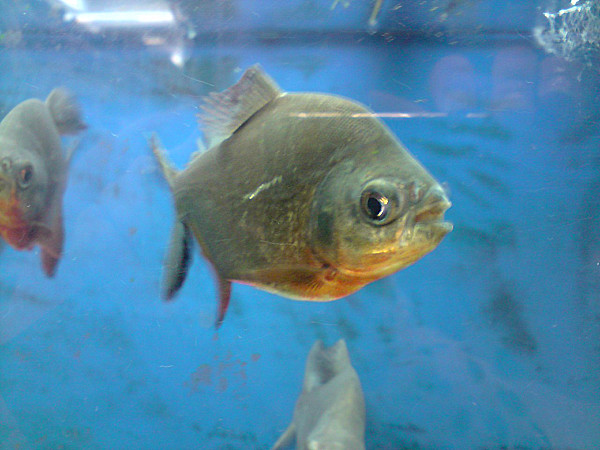In this photograph, we see an aquarium setting with a blue water background, accentuated by some black specks and a faint splash of light blue at the top right. The central focus is a small fish exhibiting a blend of colors—golden body with silver accents, and a hint of yellow around the jaw area. This fish is positioned prominently in the center, its body turned slightly to the right while facing forward, displaying notable fins on the top and back. The aquarium lighting creates reflections on the glass and illuminates the scene from the top left. To the left of the main fish, another similar fish swims towards the viewer. Below them, a third fish is partially obscured and slightly blurred. The overall ambiance suggests a calm underwater environment, captured in a precise moment of natural interaction among the three fishes.